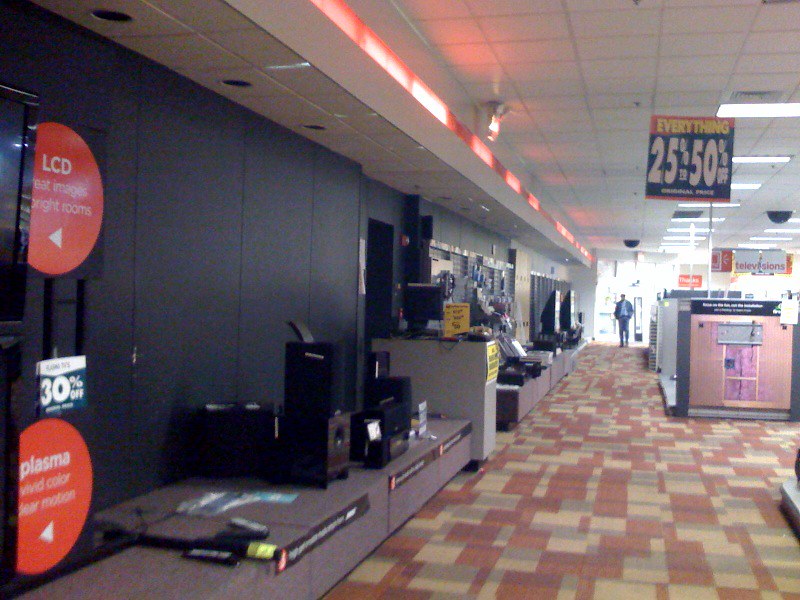The image depicts an electronics store with a white ceiling and a distinct red strip near an overhang area on the wall. Prominently, a blue sign announces a sale, offering discounts of 25% to 50%. To the left, a black wall displays various electronic items, partially cut off at the image's edge. Visible are bits of TV screens with orange signs indicating "LCD" and "plasma," alongside black speakers and a range of other electronics further back.

On the right side of the image, a capped aisle end features a brown area with gray and red elements underneath, though the specifics are unclear. Above this area, a sign labeled "Television" is visible. The floor has a retro design, composed of red, yellow, and green squares arranged in a patterned carpet. In the background, a person in a suit is seen entering the store.